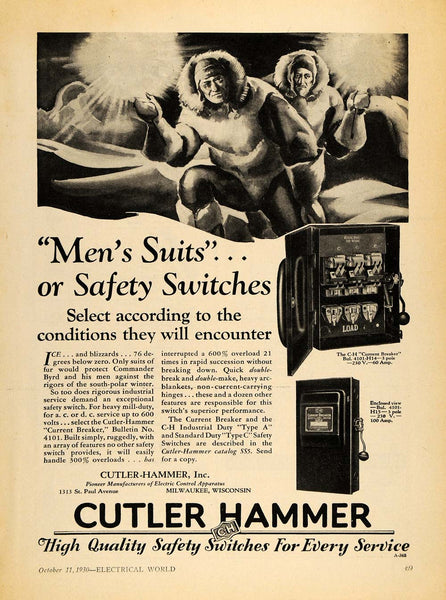This image appears to be an advertisement for Cutler Hammer, showcasing their high-quality safety switches. The advertisement, seemingly taken from an old newspaper or magazine with a yellow-brown tint, features a top section depicting a photograph of two men dressed in heavy outerwear with fur-lined hoods, traversing an icy landscape while carrying devices emitting bright light. Below this visual is the slogan, "Men's suits or safety switches. Select according to the conditions they will encounter." The ad includes images of the safety switches on the right, with columns of text that are too small to read. The bottom of the page prominently displays the company name, Cutler Hammer, with the tagline, "High quality safety switches for every service."